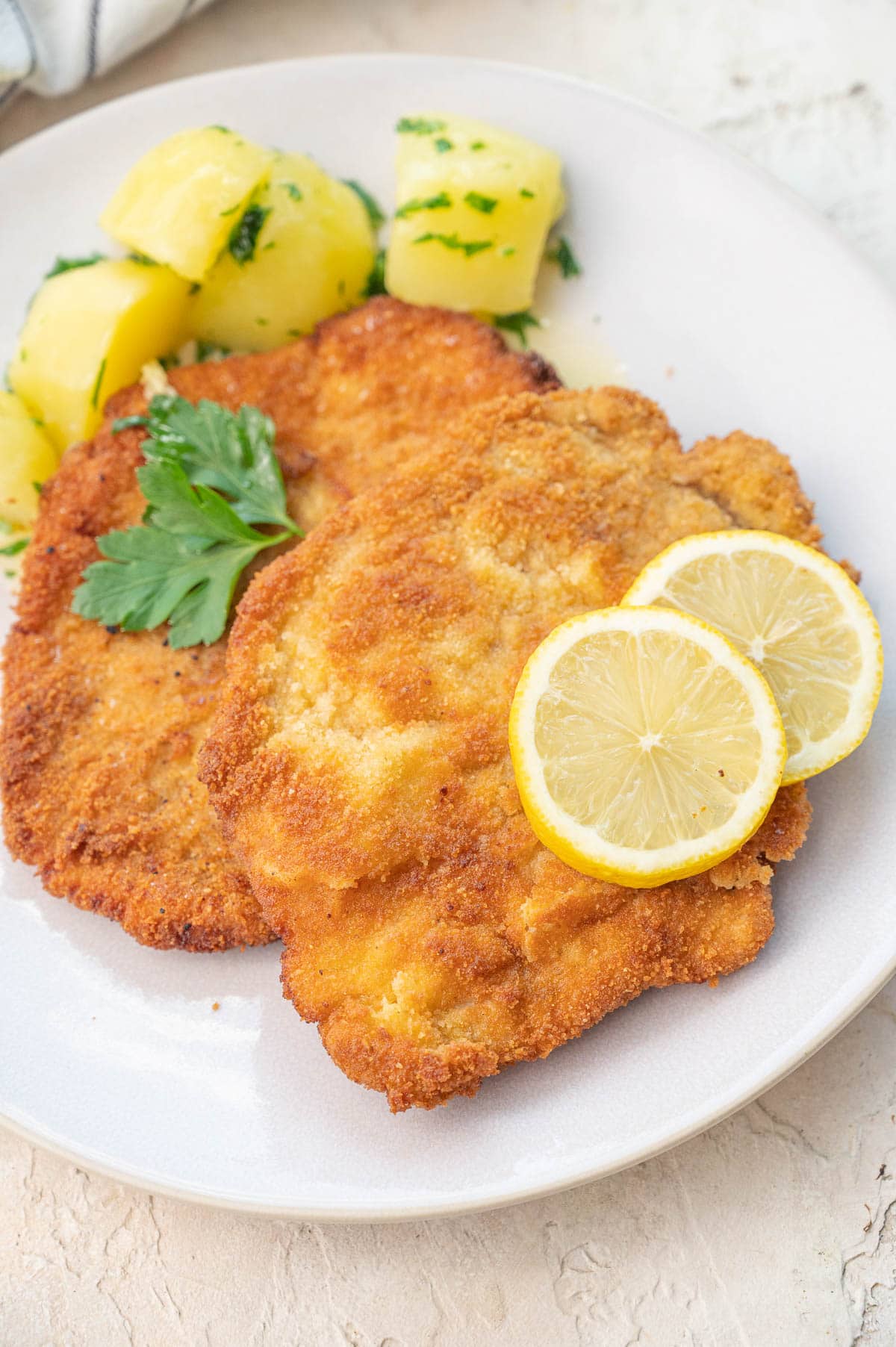The image is a color, overhead photograph of a white ceramic plate of food situated on a textured white tabletop. The main dish consists of two oval-shaped pieces of breaded and fried meat, likely Wienerschnitzel, which are a light brown color. One piece of schnitzel is garnished with two slices of lemon, while the other has a sprig of parsley or cilantro on it. In the upper left section of the plate, there are cut-up, peeled, and roasted potatoes also garnished with a sprinkle of green parsley or cilantro.